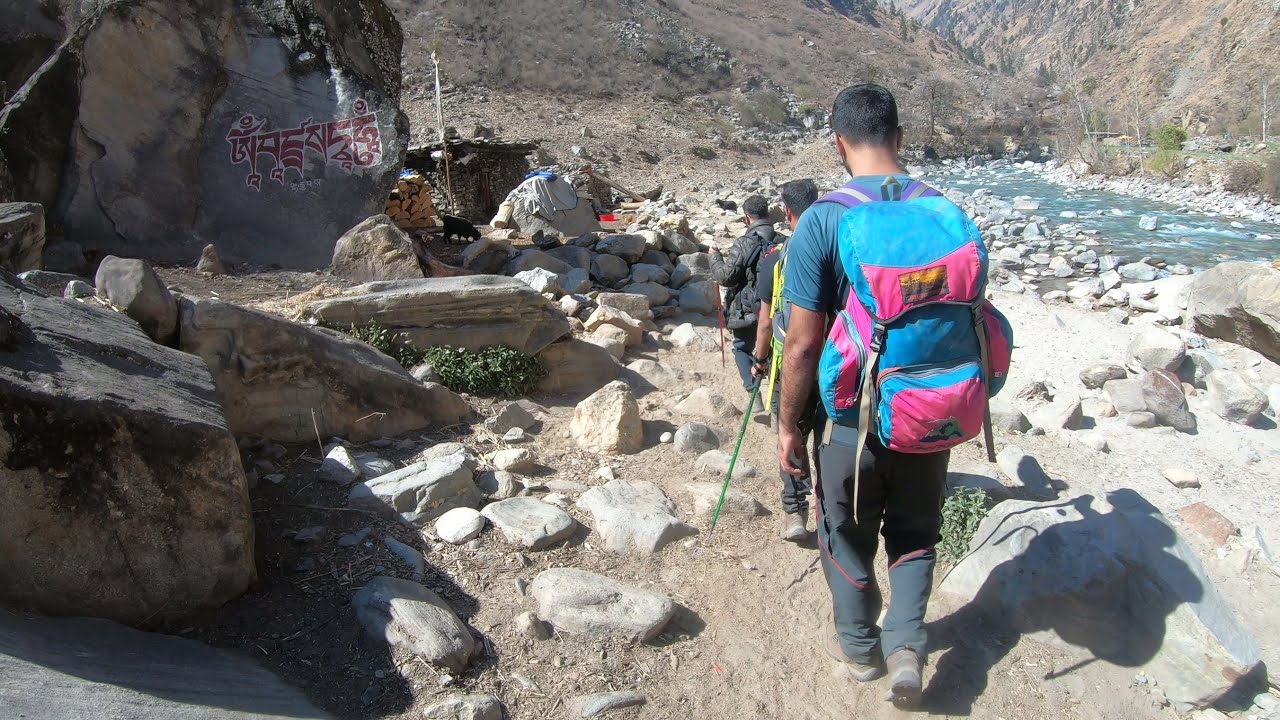In this image, we see a clear outdoor adventure scene featuring a group of hikers navigating a rugged walking trail. The trail is rocky and sandy, bordered by jagged rocks on the left and a river with a few rapids on the right. At the center of the photograph, four men are walking in line, each equipped with large backpacks and hiking gear. The first hiker closest to the camera is distinguishable by his fully packed blue and pink backpack, blue t-shirt, black pants, and hiking boots. They are heading toward a small camp with a hut made from stacked rocks and a wooden roof constructed from tilted logs. 

In the background, distant mountains and cliffs frame the scene, indicating they are in a canyon or ravine. Despite an ambiguous script appearing in the upper left corner (suggesting Middle Eastern lettering, possibly superimposed on the image), the image primarily focuses on the natural environment and the hikers. The colors in the scene range from earthy browns and tans to touches of green, blue, purple, pink, white, and yellow, all under the clear light of a sunny day. This vivid depiction situates the viewer directly in the middle of nature, capturing the essence of a mid-day hike through a remote, picturesque landscape.